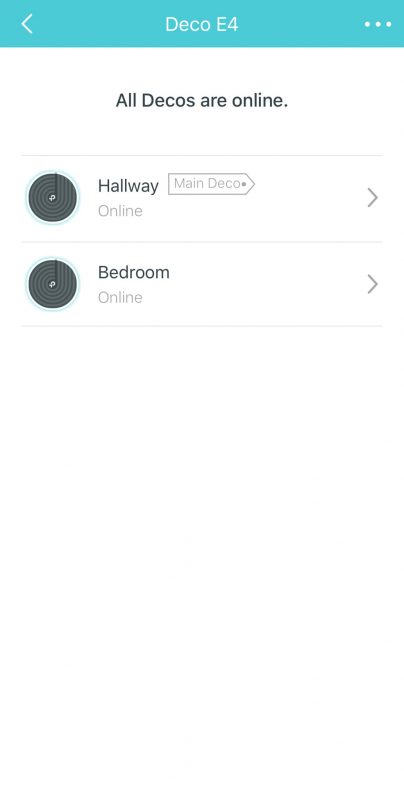The image, captured from a smartphone screen, depicts a user interface within a mobile application. 

At the very top, a teal rectangular bar spans the entire width of the screen. On the far left side of this bar, there is a left-pointing arrow. Centrally aligned within the bar, bold text reads "Deco E4" with a capitalized "E." To the right of this text, there are three horizontal dots arranged in a line, indicating a menu option for additional settings.

Below the teal bar, the background of the entire screen is white. At the top in black text, it states "All Decos are online." Just underneath this text, there are two identical black icons on the left side of the screen. Each icon is a black circle with a white dot in the center, encircled by a teal outline.

The first icon is labeled "Hallway." To the right of this label, there's a small flag-like pointer indicating "Main Deco." Directly below this, it says "Online." At the far right end of this row, there is a right-pointing arrow.

The second icon is labeled "Bedroom." Below this, it also declares "Online." Similar to the first row, there is a right-pointing arrow at the far right end of this row.